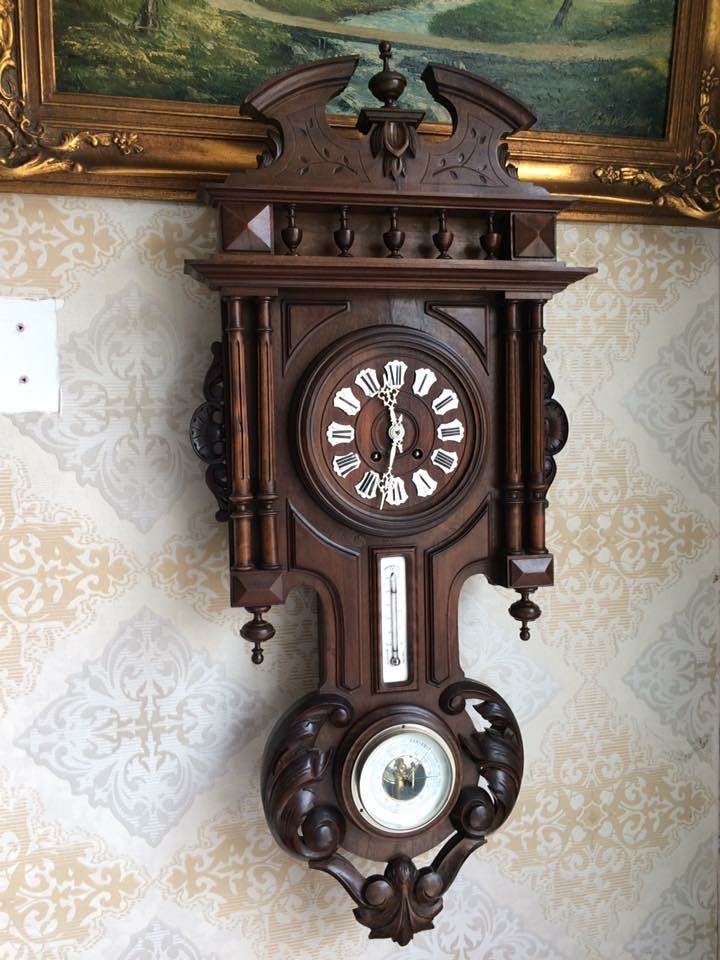The photograph, captured in portrait orientation using natural daytime lighting, showcases a close-up of an ornate, antique clock mounted on an indoor wall. The clock is meticulously crafted from wood, with intricate carvings that highlight its vintage aesthetic. Below the main clock face, a traditional glass vial thermometer is affixed, complementing the historical charm of the timepiece.

The clock face features Roman numerals, each elegantly displayed on small white tiles with crisp black lines. The clock's hands, made of white metal, are limited to an hour and a minute hand, adding to its simplistic elegance. The time is precisely depicted as 11:33, with the minute hand positioned just past the half-hour mark and between the six and seven, while the hour hand lies between eleven and twelve.

Adding to the photograph's richness, an ornate gold-framed painting sits directly above the clock. The frame is decorated with elaborate relief work, a portion of which is visible in the image, with the clock overlapping onto the bottom part of the frame, creating a layered and sophisticated visual composition.